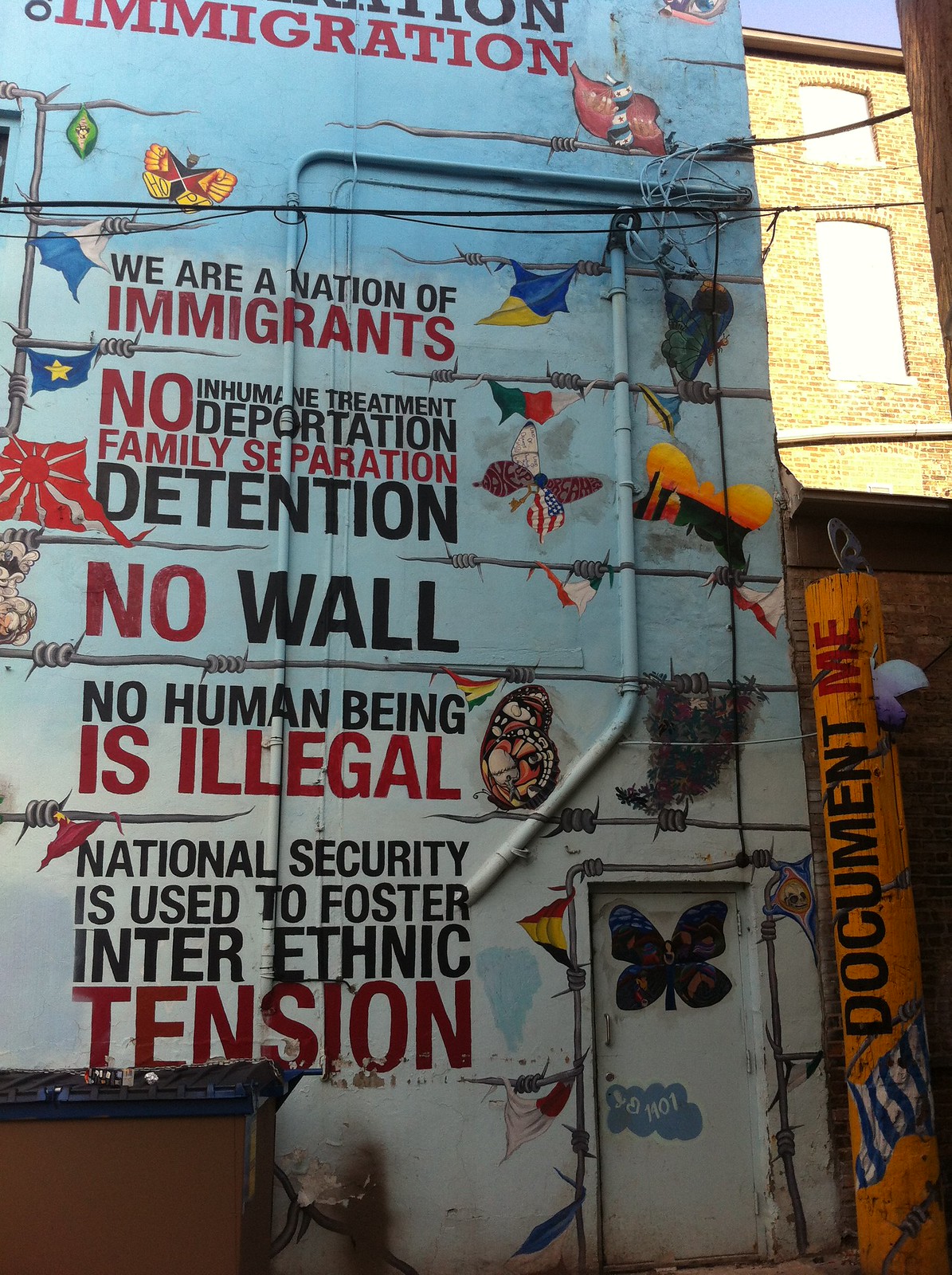The image depicts a narrow alleyway featuring a large mural painted on the exterior wall of a building. The mural, which spans more than two-thirds of the image from left to right, is set against a backdrop of a cloudy blue sky. The wall itself is worn and weathered, with pipes and wires visible along its surface. Central to the mural is the word "Immigration" in bold red lettering at the top, followed by the statement, "We are a nation of immigrants," accompanied by various fluttering butterflies with American wings and national flags.

The mural contains powerful messages in black and red text, including "No inhumane treatment," "No deportation," "No family separation," "No detention," "No wall," and "No human being is illegal." Additionally, it states, "National security is used to foster inter-ethnic tensions." These lines of text are interspersed with horizontal pieces of barbed wire, symbolizing the barriers faced by immigrants.

On the far right of the mural, there is an orange vertical strip on the brick building bearing the words "document MF," and the text "heart 1101" appears at the bottom of the mural. Above the mural, in the upper right corner, there is a gap between two buildings, revealing another brick building with bricked-up windows. One can also see an old, tattered door with a shamrock, indicating long-term disuse. The overall scene captures a poignant representation of immigration issues within a tight alleyway setting, seamlessly blending artistic elements with socio-political commentary.